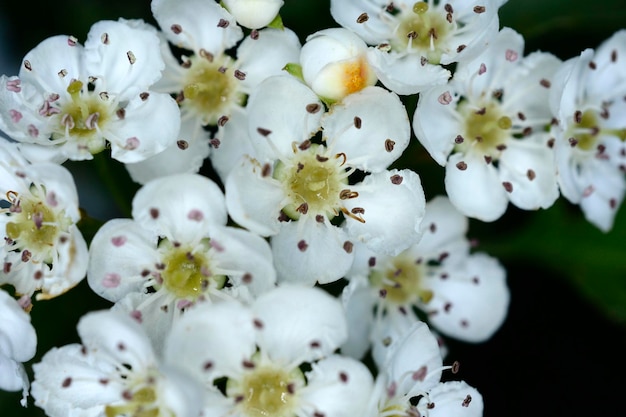This is a highly detailed close-up photograph of several white flowers, likely apple blossoms, against a dark green and blurred background. Each flower predominantly features five to six white petals, which are adorned with tiny dark purple or black spots—mostly two per petal, though this varies slightly. The centers of these flowers are a lime green to yellow color, with brownish and purplish tentacles-like structures—pistils—protruding, holding the pollen. Some flowers also exhibit faint pinkish to purplish hues, suggestive of either additional floral parts or an overlaid moth-like element. In addition, there are a couple of flowers within the cluster that have yet to unfurl their petals, remaining in a budded state. Some green leaves are partially visible, adding to the lush appearance of the floral composition. Overall, the image exudes an impression of nature's beauty through macro photography, focusing meticulously on the intricate details of the blossoms.